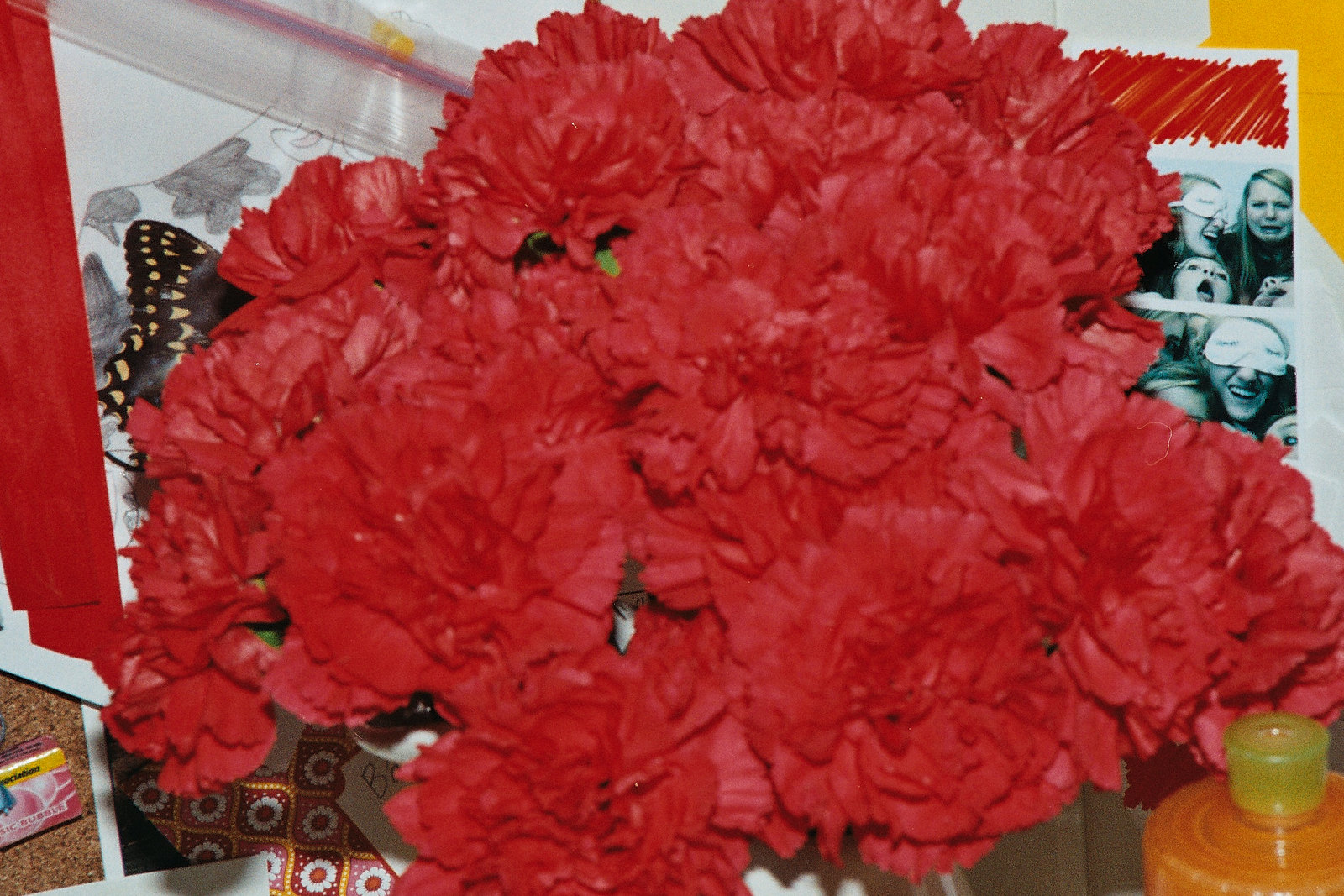In this detailed photograph, the central focus is a large, vibrant bouquet of bright red roses, tightly bundled together and fully bloomed, creating an eye-catching floral arrangement that dominates the center of the image. Surrounding this lush display, various details add depth to the composition. On the right-hand side, there are two black-and-white photo booth strips depicting a group of four women with light skin and long blonde hair, capturing playful and expressive moments; one woman sports a sleeping mask and smiles, while another exhibits a sad expression, and a third has an awe-struck look. Among the intricate surroundings, in the top left corner, a subtle monarch butterfly peeks out, partially hidden, while the bottom left showcases a repetitive gift wrap. The bottom right corner features a small candle or possibly a glass for drinking, resting on an orange surface. These elements are set against a backdrop suggesting a creative space with scrapbook art, colored drawings, and assorted materials lying on what appears to be a brown carpet.